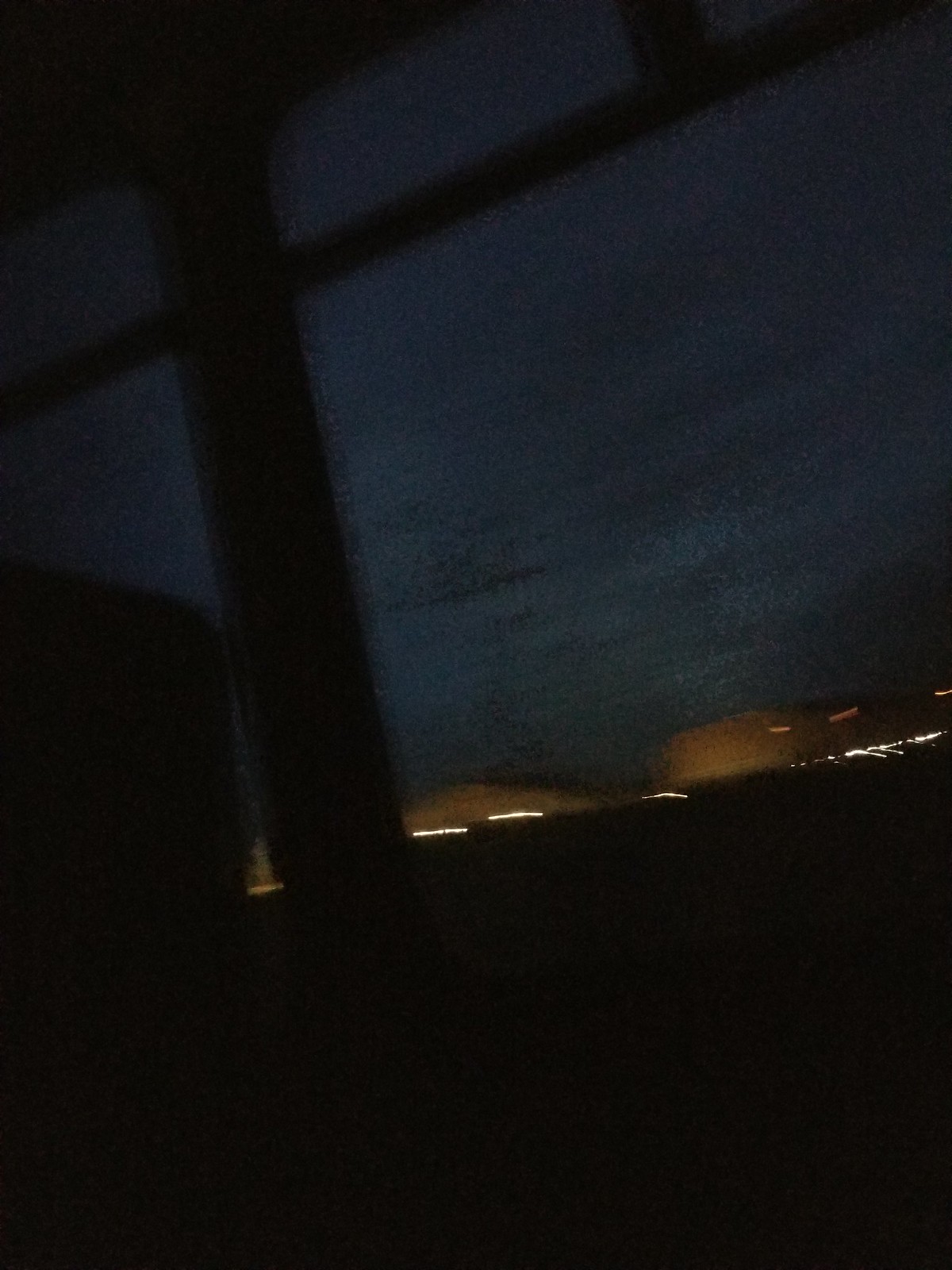The image depicts a very low-quality, blurry photograph taken at night. It appears to have been shot from inside a large vehicle, likely a Greyhound bus, as the outline of a bus window and a seat in silhouette are visible in the foreground. The dark blue, almost black night sky dominates the background, marred by occasional dark spots. The bottom of the picture is enveloped in dense darkness, rendering it flat and one-dimensional.

In the distance, faint lights illuminate the scene, with a noticeable cluster towards the right. Far off the road, two large, white-colored buildings stand out, highlighted by lights along their roofs or sides. These structures are situated next to each other but remain unconnected, contributing to the eerie yet intriguing atmosphere captured in this nocturnal snapshot. The image suggests motion, likely due to the bus traveling swiftly along a freeway, which accounts for the blurred quality.